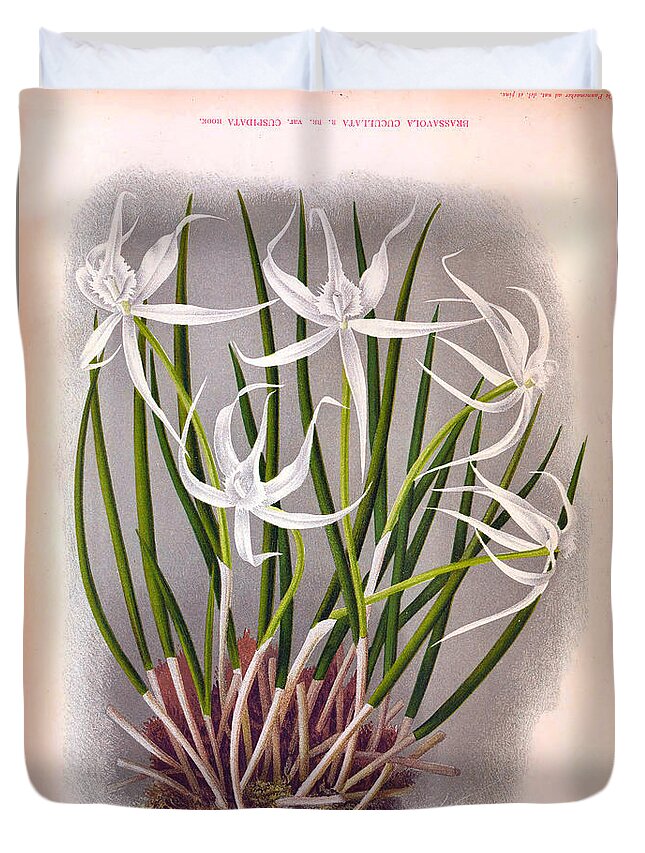This image is a detailed depiction of a flowering plant, likely a scientific or botanical illustration, superimposed onto a sales mock-up for a comforter. The background consists of a beige or pinkish hue with wavy borders that give the appearance of a bag. The central subject is a plant with multiple green stems, ranging from dark to light green, and brown and white stems at the base. The plant features five large white blooms, each with thin, long petals that suggest a six-petal arrangement, reminiscent of lilies. Each flower centers around a small, protruding white bulb or cone shape. The base of the plant includes light cream-colored tubular structures and some dark red, spiky leaves. There is unreadable text at the top, possibly in Latin, indicating the scientific name "Brassavola cuculata." The image conveys a vintage, scientific artistic style and also functions as a potential bedding advertisement, with the floral illustration likely intended to showcase the design on a comforter or duvet cover. White pillows are visible at the top of the scene, enhancing the bedding context.